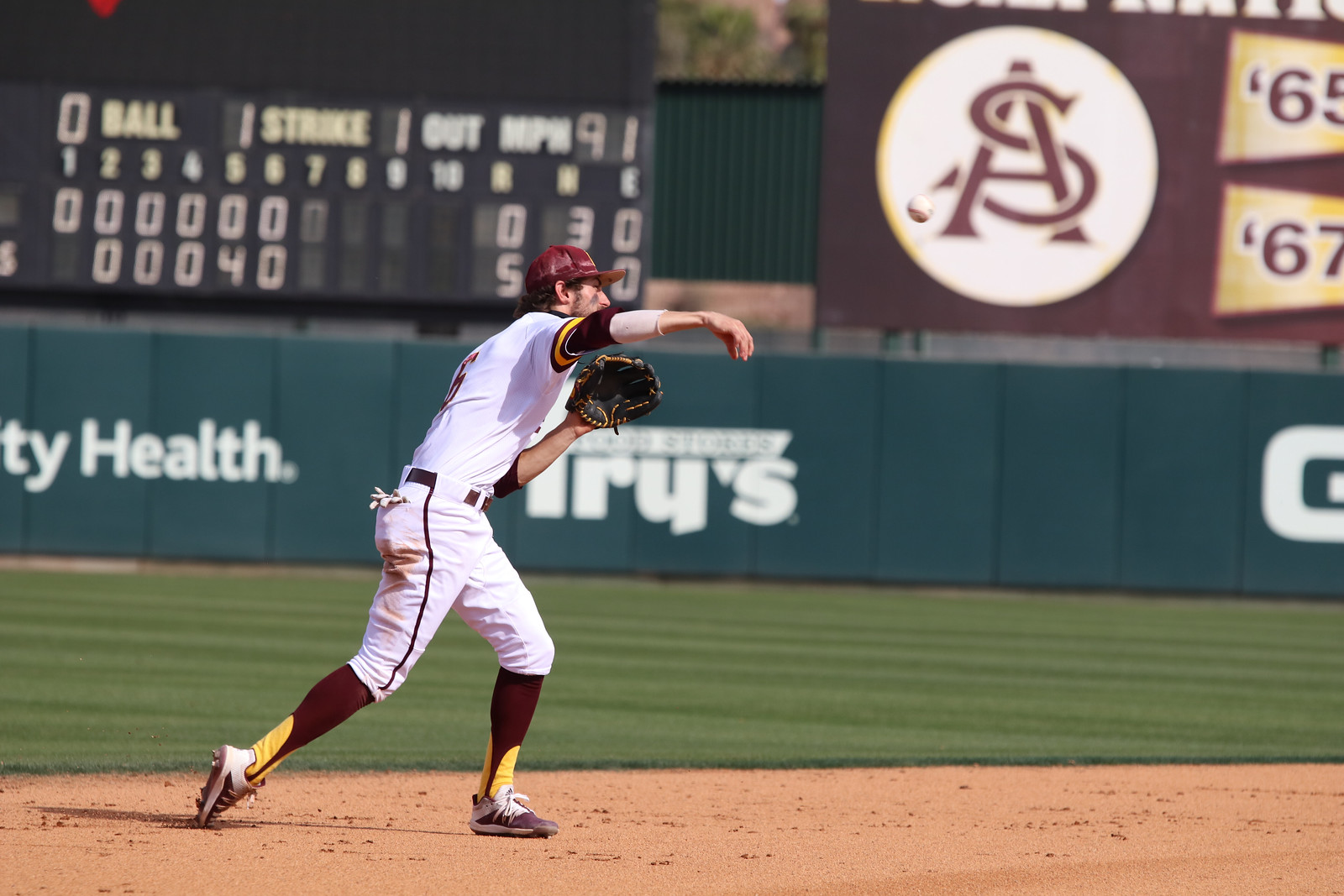In this detailed photograph from a daytime baseball game, we see an infield player executing a dynamic throwing motion. The player is outfitted in a pristine white jersey and pants, complemented by burgundy and gold underclothing and a matching burgundy and gold hat. His ensemble includes brown and yellow socks, white cleats, and a baseball glove on his left hand while his right hand is mid-throw. The scene is set against a meticulously mowed green outfield, bordered by a barricade adorned with various sponsorship logos, including "PY Health," "AROs," and more. To the left above the wall, the scoreboard displays the game status with zero balls, one strike, and one out, alongside the team's score and more numbers indicating game progress. Additionally, a brown signboard with a circular logo featuring "ANS" and the numbers 65 and 67 is visible on the right-hand side, behind which stands a green building and some trees. The bright sunlight bathes the field, highlighting the vivid colors and details, capturing the essence and energy of the game.